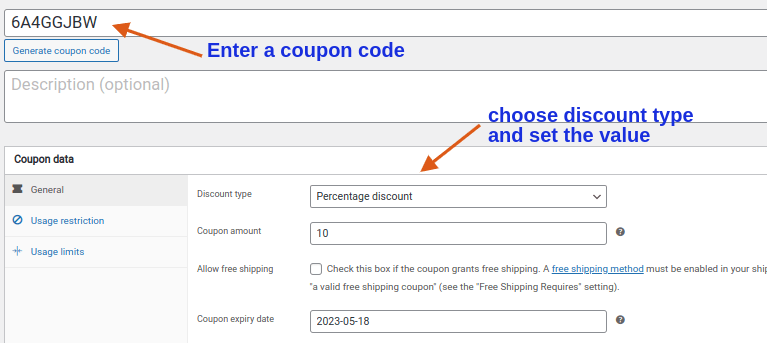A comprehensive screenshot of an online sales management interface for small businesses. The screen displays the setup process for discount coupons. At the top, a text box contains the code "6A4GGJBW," highlighted by a red arrow. Next to the arrow, blue text reads "Enter a coupon code." Below, a button labeled "Generate Coupon Code" suggests it can create a random text string for the coupon.

Further down, a text box labeled "Description optional" is visible. Below this, a section titled "Coupon Data" features a gray bar with three tabs: "General," "Usage Restriction," and "Usage Limits," with "General" currently selected.

To the right, under "General," a dropdown menu labeled "Discount Type" is set to "Percentage Discount." A blue arrow points to this area with text advising to "Choose discount type and set the value." Beneath this, a field labeled "Coupon Amount" shows the value "10," indicating a 10% discount.

The interface includes an option to "Allow Free Shipping," with instructions to check the box if the coupon grants free shipping, although some text is clipped. Finally, the "Coupon Expiry Date" is set to "2023-05-18."